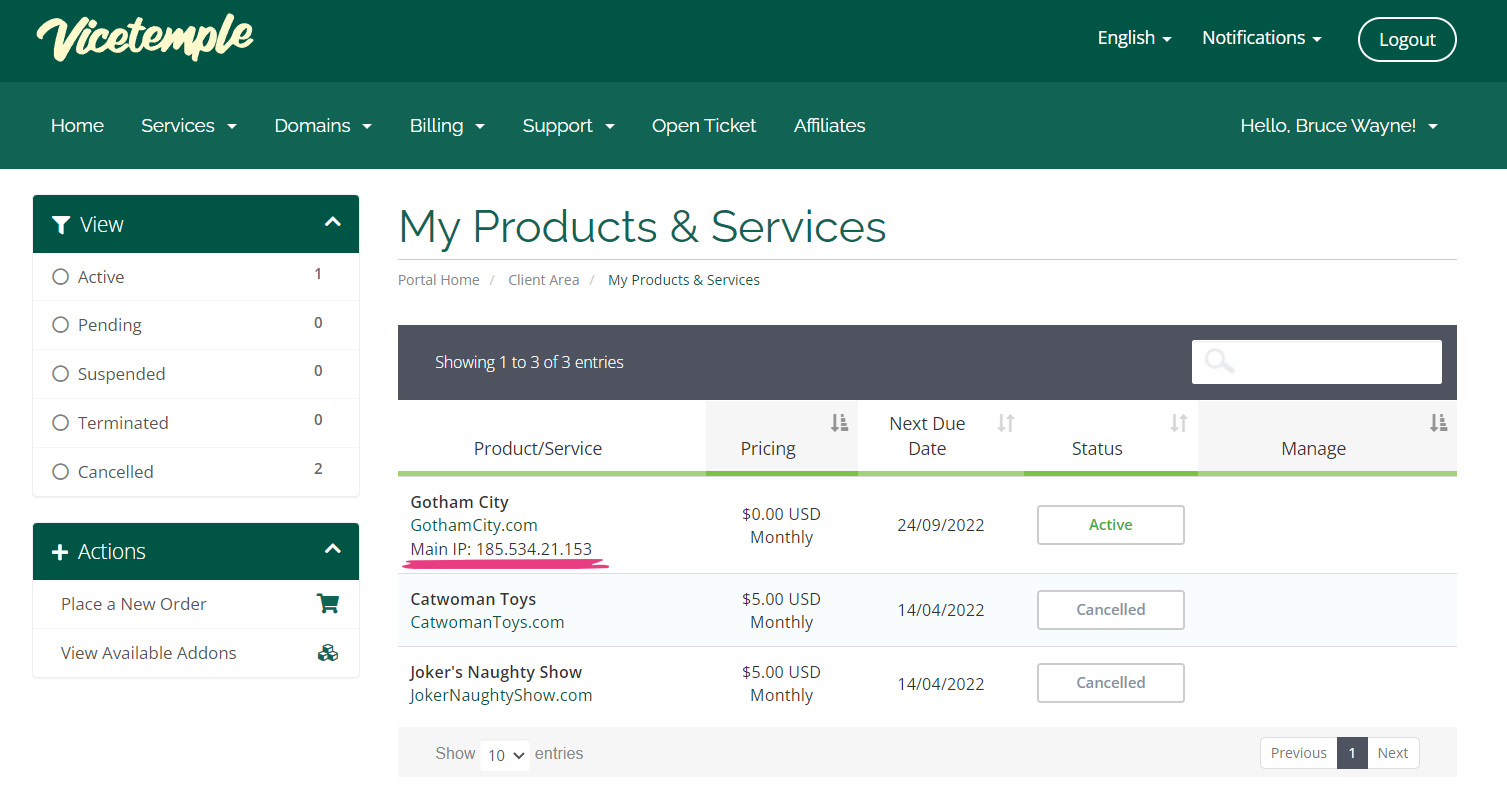This image is a comprehensive screenshot of a dashboard from what appears to be a website or web application, characterized by a landscape orientation with notable width and shallow height. 

At the very top, a dark green navigation bar spans the entire width of the image. Positioned in the top left corner is the logo for the website, "Vice Temple," rendered in a cursive-style font with text color that is either white or a very light cream yellow. On the top right, a navigation layout is presented with several options: a dropdown menu labeled "English," a "Notifications" option, and a "Logout" button. The "Logout" button is outlined in white, revealing the green background behind it.

Below this, there is a secondary navigation bar with a lighter—but still dark—green background. This bar houses multiple menu items including "Home," "Services" (with a dropdown), "Domains" (with a dropdown), "Billing" (with a dropdown), "Support" (with a dropdown), "Open Ticket," and "Affiliates." On the right end of this bar, the user is greeted with "Hello Bruce Wayne," accompanied by a dropdown menu.

The main content of the page is organized into two primary sections on a white background. The left section is a sidebar displaying various navigational and actionable items, whereas the right section presents detailed user-specific data.

Starting with the left sidebar:
- This section includes collapsible (accordion) menus.
- The first collapsible menu is titled "Active" and shows metrics such as Active (1), Pending (0), Suspended (0), Terminated (0), and Canceled (2), each prefixed with a small circle.
- The second collapsible menu is labeled "Actions" and contains options to "Place a New Order" and "View Available Add-ons," each accompanied by an icon to the right.

In the right section—the main content area of the dashboard:
- The header reads "My Products and Services."
- Directly beneath the header, breadcrumb navigation indicates the user's current page: "Portal / Home / Client Area / My Products and Services."
- Below the breadcrumbs is a dark gray bar containing white text: "Showing 1 to 3 of 3 entries," with an embedded search bar on the right.
- The primary data is displayed in a tabular format with alternating light gray rows for readability.

The table is divided into five columns: 
- "Product/Service"
- "Pricing"
- "Next Due Date"
- "Status"
- "Manage"

Three rows of user data are listed:
1. **Row 1 (Active)**:
   - **Product/Service**: GothamCity.com
   - **Main IP Address**: A string of numerical IP data
   - **Status**: Active

2. **Row 2 (Canceled)**:
   - **Product/Service**: CatwomanToys.com
   - **Status**: Canceled

3. **Row 3 (Canceled)**:
   - **Product/Service**: JokerNaughtyShow.com
   - **Status**: Canceled

Overall, the dashboard is designed to provide a detailed and organized overview of the user's products and services, facilitating easy navigation and accessibility of pertinent information.